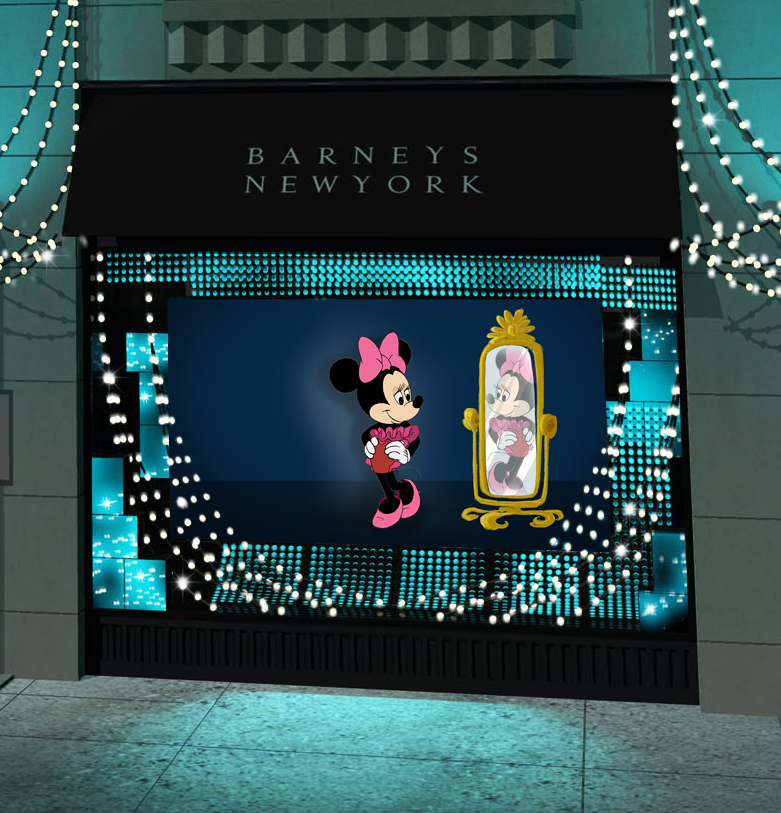This image is a detailed, artistic rendering of a storefront, specifically Barney's New York. The scene is set at nighttime, lending a dark, serene ambiance. At the top of the storefront, a black banner prominently displays the name 'Barney's New York' in gray letters. Below the banner, a large window display captures attention. Here, Minnie Mouse is depicted joyfully admiring herself in a golden-framed mirror while wearing a pink frilly dress, bright shoes, and a bow on her head. The mirror is positioned to her right.

The window display is adorned with various lights, including green and blue LEDs and cascading white string lights, reminiscent of Christmas decorations. These lights create a festive, glowing atmosphere around the display and along the building’s exterior, stretching into the top corners of the image. 

The building itself is constructed from concrete bricks, and a gray, rendered sidewalk extends in front of it, grounding the whimsical display in a more mundane urban setting. Overall, this rendered scene combines the enchanting allure of animated characters with the sophisticated urban façade of Barney's New York, illuminated beautifully against the night sky.